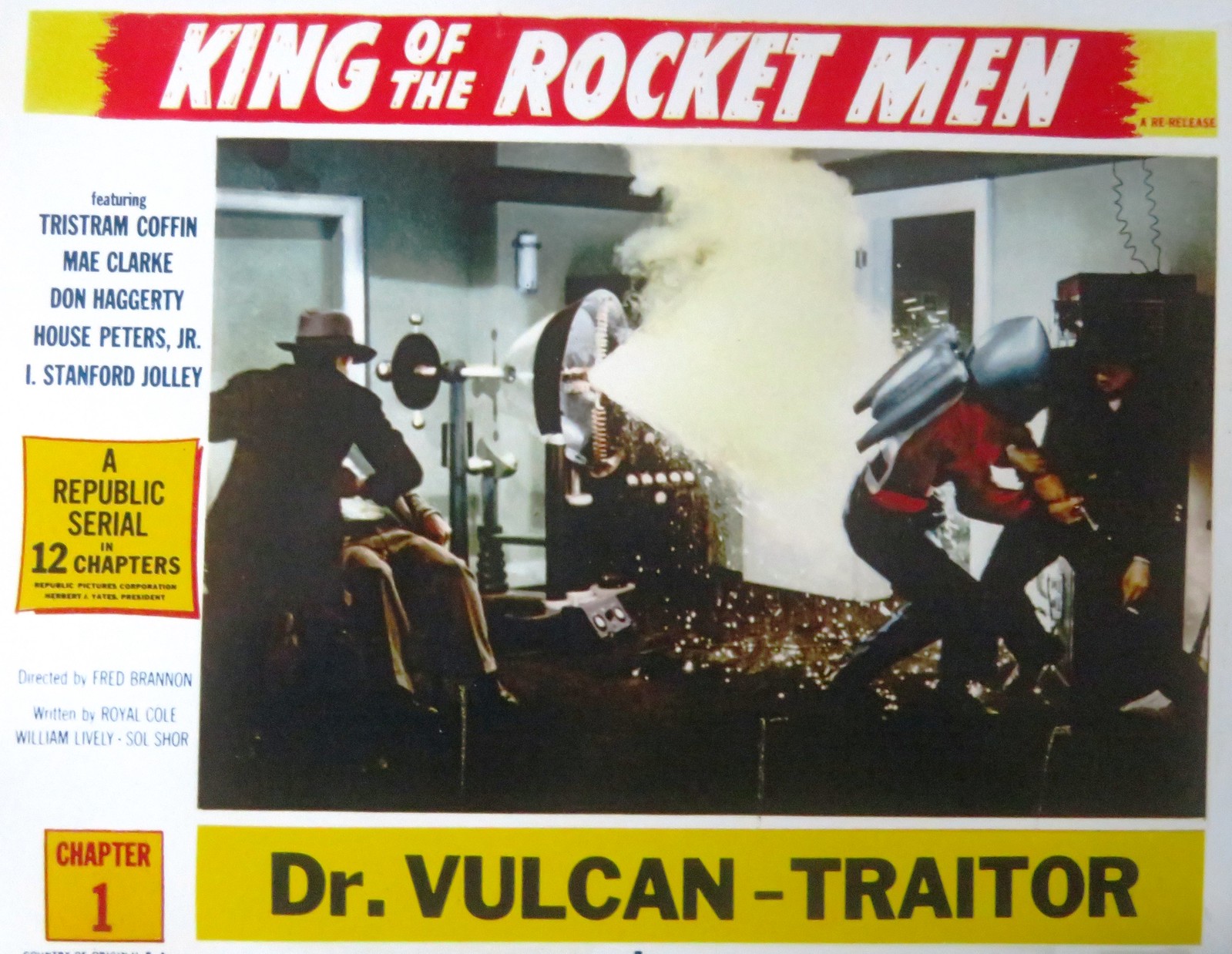This vintage movie poster for "King of the Rocket Men" features a dramatic, action-packed scene in the center, depicting a chaotic explosion with bursts of steam and sparks. In the foreground, four men are engaged in intense combat. On the left, a man in a stylish jacket and hat from the 1950s wrestles with an unseen opponent, while on the right, another man, clad in a mostly black outfit, grapples with a figure dressed in a red top, silver helmet, and equipped with a jetpack, likely the Rocket Man himself. The vivid action scene captures the adventurous spirit of the serial.

At the top of the poster, a bold red strip over a yellow background bears the title "King of the Rocket Men" in white text, with a note about its re-release. Flanking this central title, yellow edges frame the strip. The left side of the poster features a vertical column listing the cast: Tristam Coffin, Mae Clarke, Don Haggerty, House Peters Jr., and I. Stanford Jolly. Below this cast list, another section credits the film as "A Republic Serial in 12 Chapters," directed by Fred Brannan and written by Royal Cole and William Lively.

At the very bottom, a yellow rectangle boldly announces, "Dr. Vulcan, Traitor," in black text, set against the backdrop of a climactic scene from the serial’s first chapter, as indicated by a similarly styled yellow box highlighted with the red text "Chapter 1."

Overall, the poster's muted tones and dynamic design effectively capture the essence of this classic serial adventure, inviting viewers into the thrilling world of "King of the Rocket Men."